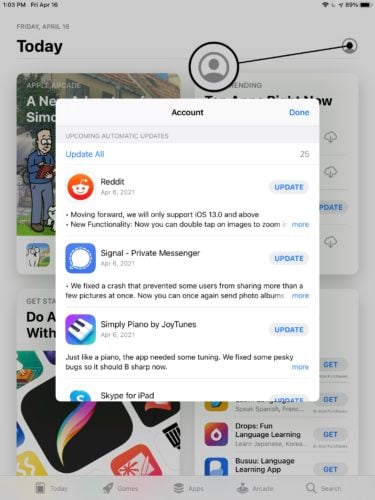This image showcases the App Store interface on an iPhone, focusing on the profile picture icon, which serves as a portal to the account settings. By clicking on this icon, users can access a list of apps associated with their account, including those pending updates. The highlighted section indicates upcoming automatic updates for several applications: Reddit, Signal Private Messenger, Simply Piano by Joytunes, and Skype for iPad. 

Each app features its recognizable icon and detailed update notes:
- **Reddit**: "Moving forward, we will only support iOS 13 and above. New functionality: now you can double-tap on images to zoom."
- **Signal Private Messenger**: "We fixed a crash that prevented some users from sharing more than a few pictures at once. Now you can once again send photo albums."
- **Simply Piano by Joytunes**: "Just like a piano, the app needed some tuning. We fixed some pesky bugs, so it should be sharp now."
- **Skype for iPad**: General improvements and bug fixes for better performance.

In the background, the interface also displays some recommended apps for the day, providing users with suggestions for new downloads and discoveries.